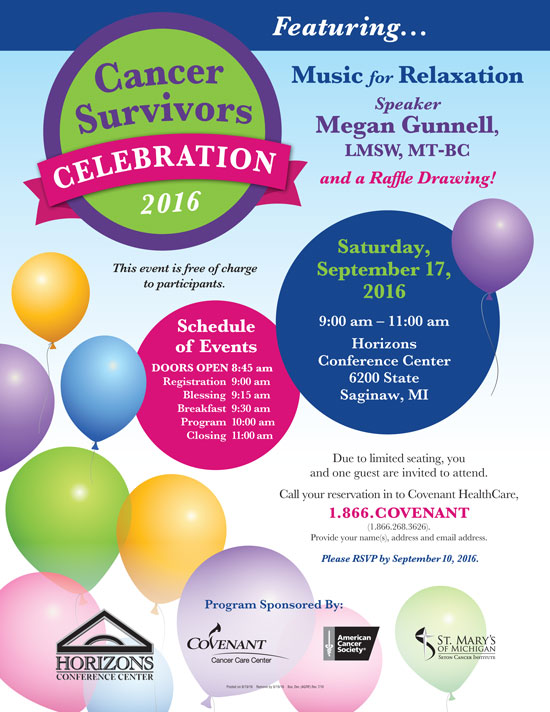The image is a rectangular poster advertising a "Cancer Survivors Celebration 2016." The background is predominantly light blue with scattered balloons in various colors including blue, yellow, and green, predominantly in the bottom left-hand corner. The poster features multiple colored text and circled text areas, giving it a cheerful and inviting appearance.

At the top, the poster prominently announces "Cancer Survivors Celebration 2016." It highlights that the event will feature music for relaxation, with a speaker, Megan Gunnell, LMSW, MTBC, and includes a raffle drawing. The event is free of charge for participants and is scheduled for Saturday, September 17th, 2016, from 9 a.m. to 11 a.m. at the Horizons Conference Center, located at 6200 State Street, Saginaw, Michigan.

To the left, there's a detailed schedule of events:
- Doors open at 8:45 a.m.
- Registration at 9:00 a.m.
- Blessing at 9:15 a.m.
- Breakfast at 9:30 a.m.
- Program at 10:00 a.m.
- Closing at 11:00 a.m.

The poster also includes a note about limited seating, inviting each participant to bring one guest. Reservations can be made by calling Covenant Health Care at 1-866-COVENANT (1-866-268-3626), with contact details such as name, address, and email address. Participants are asked to RSVP by September 10th, 2016.

At the bottom of the poster, there are logos of the event sponsors, which include the Horizons Conference Center, Covenant Cancer Care Center, the American Cancer Society, and St. Mary’s of Michigan.